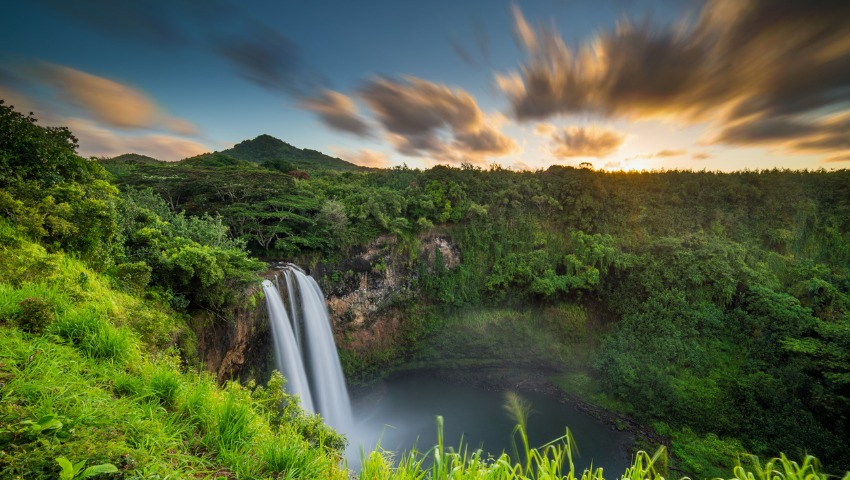The image captures a breathtaking aerial view of a lush, tropical landscape dominated by a cascading waterfall that pours into a murky, gray lagoon below. Surrounded by rocky outcroppings, the waterfall descends from the top left of the frame, with white water contrasting starkly against the rugged cliffs. The backdrop features a blend of rolling hills and dark, tree-lined mountains, creating a dramatic scene. The foreground is dotted with light green grass and vegetation, enhancing the verdant atmosphere. Above, a blue sky stretches across the horizon, interspersed with clouds that appear in motion, their dark gray centers juxtaposed with golden tips, as if caught by the setting sun. The photograph is almost panoramic in scope, exuding a 3D effect, with the motion-blurred clouds enhancing the dynamic feel of the scene.